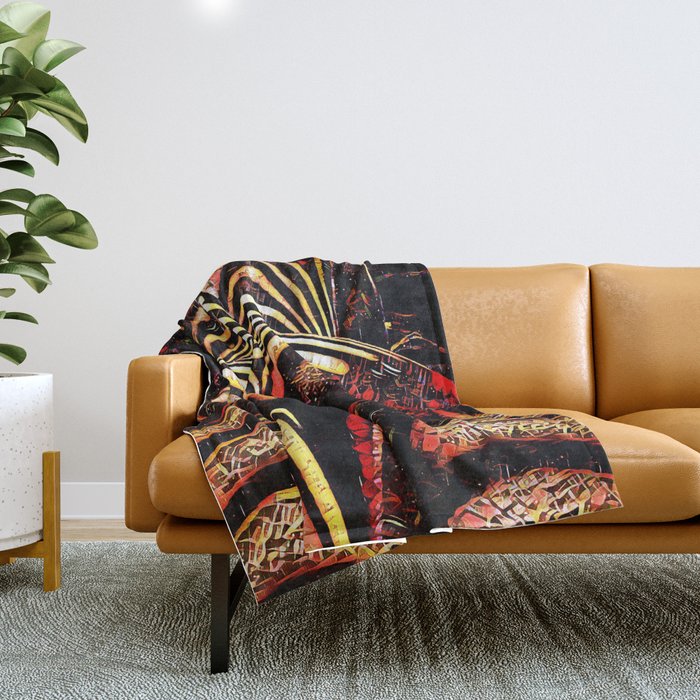In the image, a light brown leather sofa occupies the front right and center portions of the room. Draped casually over one corner of the sofa is a patterned blanket, showcasing colors in varying shades of black, red, yellow, and brown. The sofa rests on a wooden floor partially covered by a light gray, patterned rug. On the left-hand side, partially cut off but still prominently visible, stands a large cylindrical white speckled planter housing a tall green leafy plant. This eclectic arrangement presents a cozy and inviting atmosphere within the room.